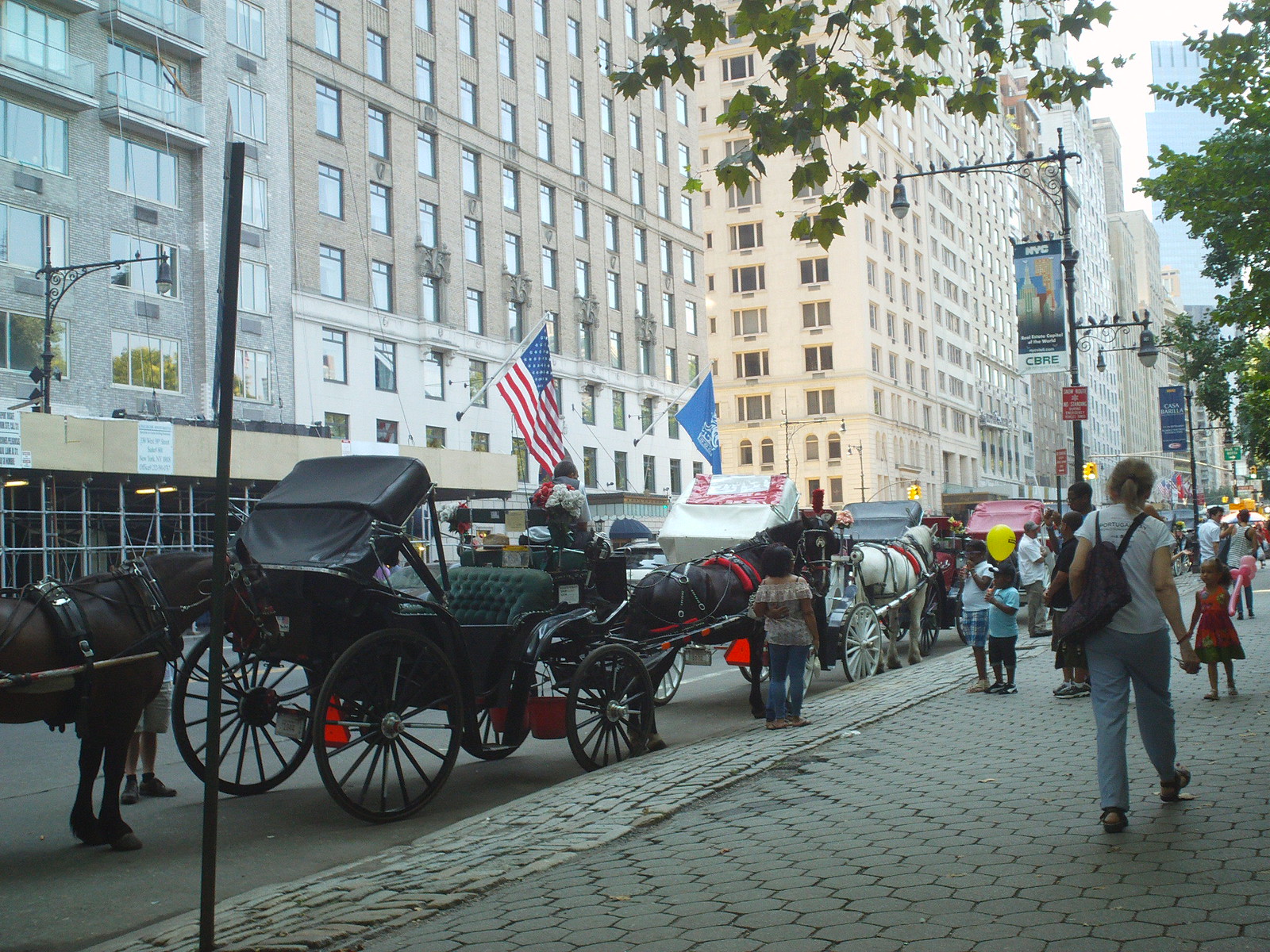In this vibrant street scene set in a bustling big city, majestic skyscrapers and towering older buildings, painted in shades of white and off-white, frame the backdrop. The photo, taken from the left, captures a sidewalk paved with unique hexagonal stone tiles. At the forefront and extending across the street are several horse-drawn carriages. Notably, a dark brown horse is hitched to a black carriage with green seats, while a stately white horse is coupled with a white carriage. 

Adding to the lively atmosphere, numerous people, including children, stroll along the sidewalk. A child clutching a yellow balloon stands out among the crowd. The scene is adorned with an array of flags; an American flag and a blue flag, likely inscribed with "NYC," are prominently displayed on nearby light posts and on buildings. Meanwhile, patches of greenery peek through in the form of leaves on partly visible trees, all basking in the glow of a bright daytime sky.

This quintessential urban vista—with its mix of old-world charm and modern-day leisure—captures a slice of city life, complete with the picturesque allure of horse-drawn carriages awaiting their next passengers.